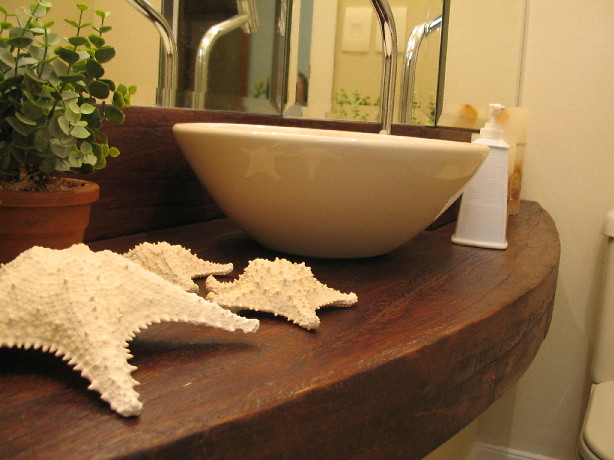The photograph captures a stylish bathroom setting. Central to the image is a thick wooden countertop with a curved edge, resembling a half oval in shape. Atop this countertop sits a cream-colored, vessel-style sink, paired with a sleek chrome faucet. To the right of the sink, there's a white ceramic pump bottle, typically used for hand soap. Partially obscured behind the pump bottle are some cream and brown objects, possibly candles, though they are out of focus. 

In the lower right corner of the image, the left edge of a toilet is visible. A white baseboard runs along the bottom of the wall, which is painted in a light beige color. The upper part of the image showcases a mirror behind the sink, reflecting houseplants, two light switches on an adjacent wall, and a glimpse of a blue wall seen through what appears to be a doorway. 

In the foreground, three large white dried starfish are arranged on the left side, adding a nautical touch. Additionally, a houseplant in a terracotta pot with many stems and round leaves is present on the left, contributing to the bathroom's serene and decorative ambiance.